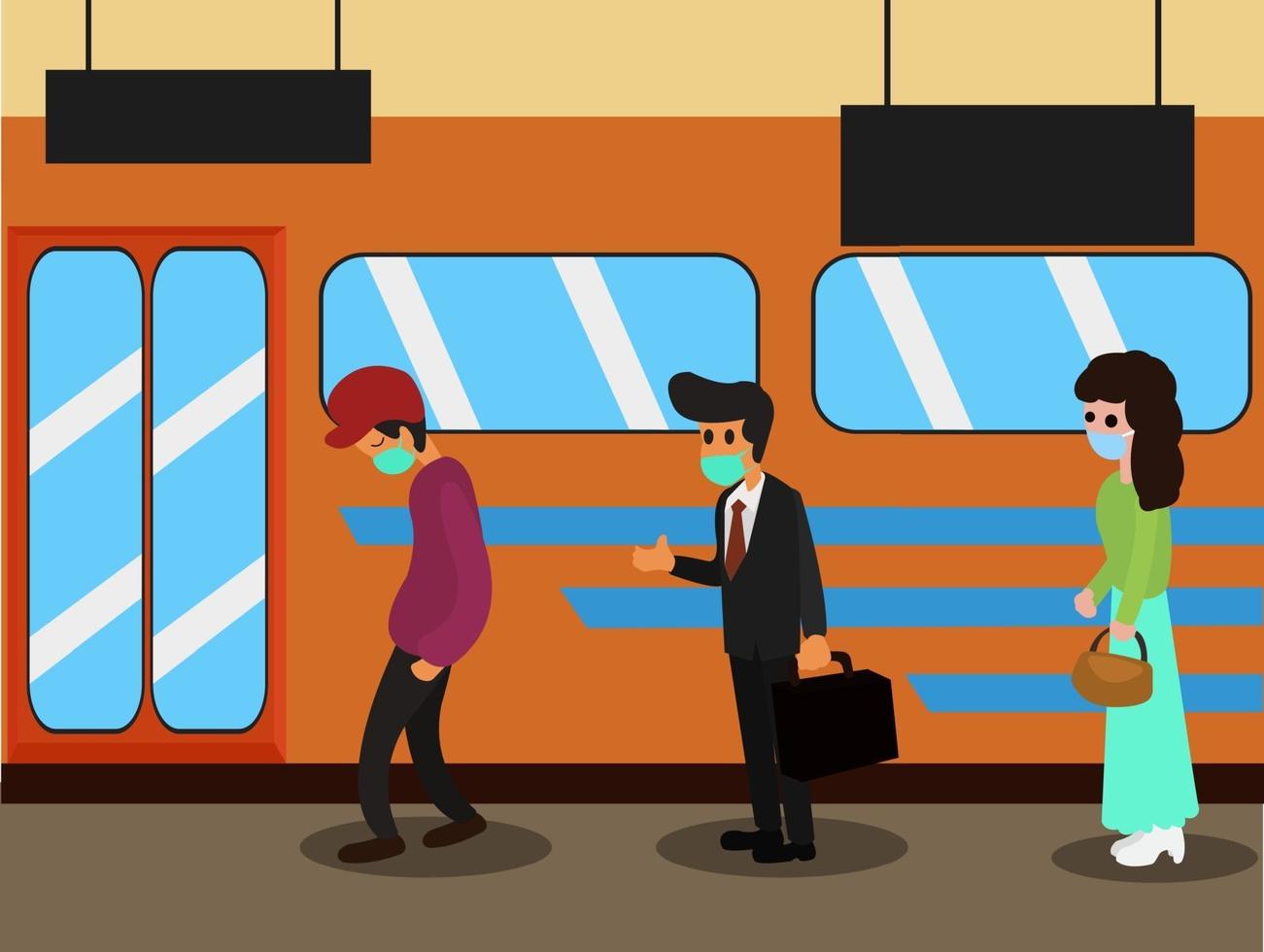This vibrant and colorful cartoon illustration depicts a scene at a subway station, seemingly set during the COVID-19 pandemic. Three masked individuals are lined up, each standing on social distancing markers on the platform. The train, painted orange with blue windows, has pulled into the station and has its doors open, ready for boarding. The first person in line is a boy with a red baseball cap, black pants, a purple shirt, and his hands in his pockets. He appears to be looking down, perhaps in disappointment. Behind him stands a businessman clad in a black suit, a white button-down shirt, and a maroon tie. He carries a black briefcase in one hand and inexplicably holds out his other hand. Lastly, a woman with long black hair waits at a distance. She wears a blueish-green skirt, a green sweater, white shoes, and holds a tan pocketbook. Despite a few signs above the train, the information on them is not visible. This image captures a moment of everyday life adjusted for pandemic safety protocols, highlighting the masks and social distancing measures in place.